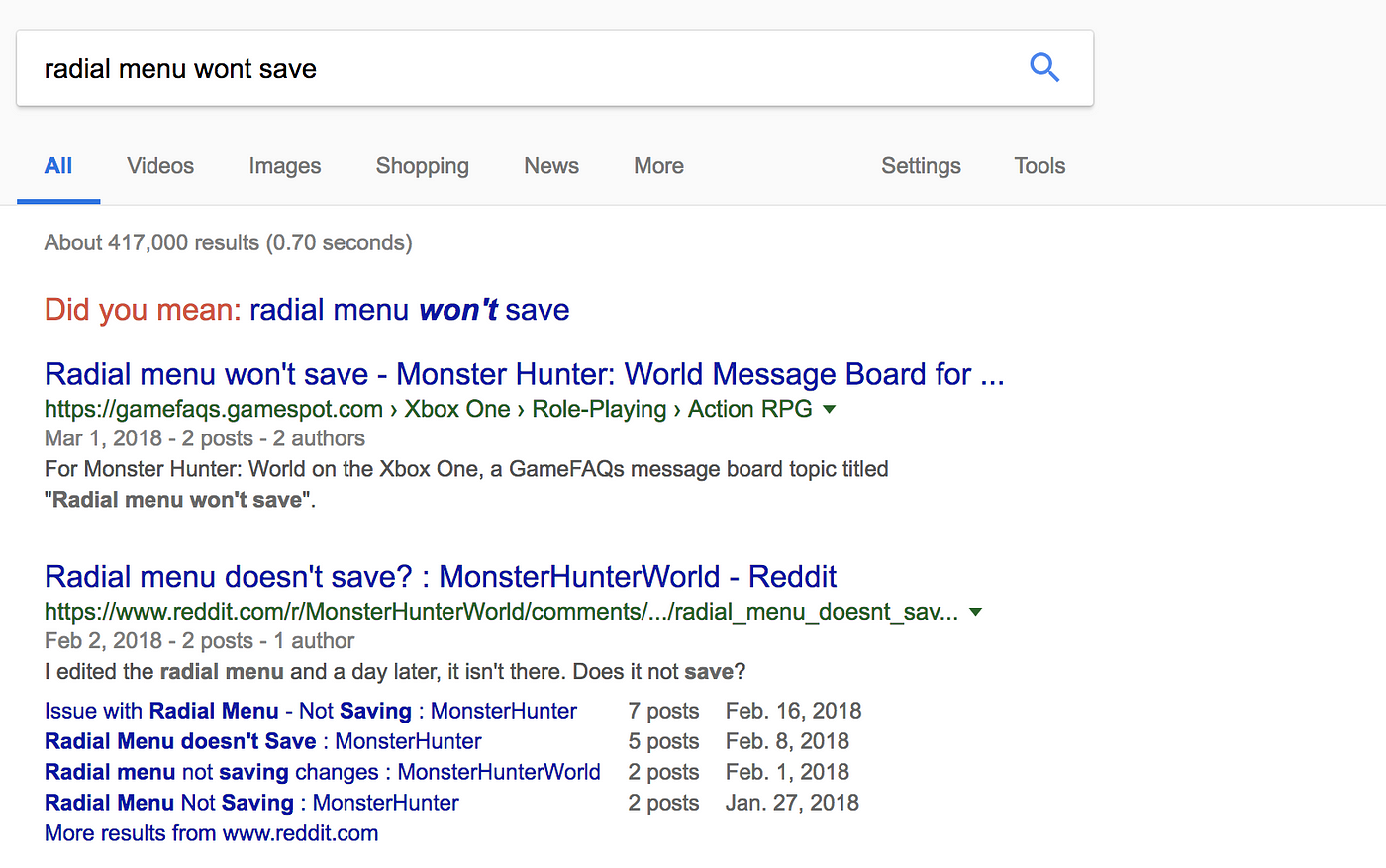The image is a horizontally-oriented rectangle featuring a user interface screenshot resembling a search engine results page. The top quarter of the image is dominated by a light gray banner, within which there is a white search box. Inside the search box, in black text, it reads "radial menu won't say," accompanied by a search icon on the far right.

Directly below the banner, a navigation bar provides various filter options: "All," "Videos," "Images," "Shopping," "News," and "More," starting from the left and extending towards the middle. On the right side of this navigation bar, "Settings" and "Tools" are listed. The "All" option is highlighted in blue and underlined, indicating it is the selected filter.

Further down, the page displays a summary in small text stating "About 417,000 results (0.70 seconds)." Below this, there is a suggestion in red text reading "Did you mean:" followed by "radial menu won't save" in blue text with an apostrophe included.

Two search results are then displayed. The first result reads, "radial menu won't save - Monster Hunter World Message Board 4…" and the second one says, "radial menu doesn't say? — Monster Hunter World Reddit."